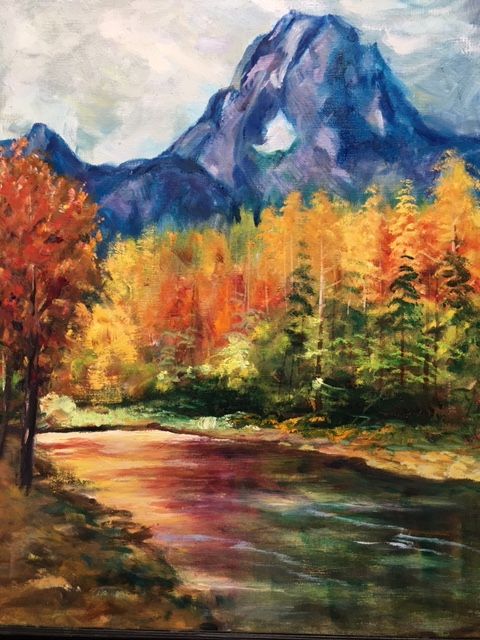This painting captures a serene autumn riverbank scene, rich in detail and color. Dominating the foreground is a singular tree with vibrant orange foliage, standing on a patch of decaying fall grass colored in varying hues of green and yellow. The river, flowing from the mid-ground towards the foreground, reflects the surrounding autumnal colors—a gradient of oranges, reds, yellows, and transitioning into darker greens near the viewpoint. The river thus mirrors the foliage on its banks, enhancing the seasonal atmosphere.

On the far bank, dense clusters of trees extend towards the horizon, their leaves exhibiting a palette from deep greens to lighter greens interspersed with vivid reds and oranges. The backdrop features a majestic blue mountain, which stands out prominently with patches of white, possibly indicating snow or a cave-like formation at its center. Above, the sky is a blend of light gray and white clouds, suggesting a cloudy day with subtle sunlight peeking through, casting a gentle glow reflected on the water’s surface, infusing hints of yellow into the scene.

This artistically rendered landscape, possibly inspired by the likes of Monet, beautifully captures the essence of an autumn day with its harmonious blend of colors and natural elements.